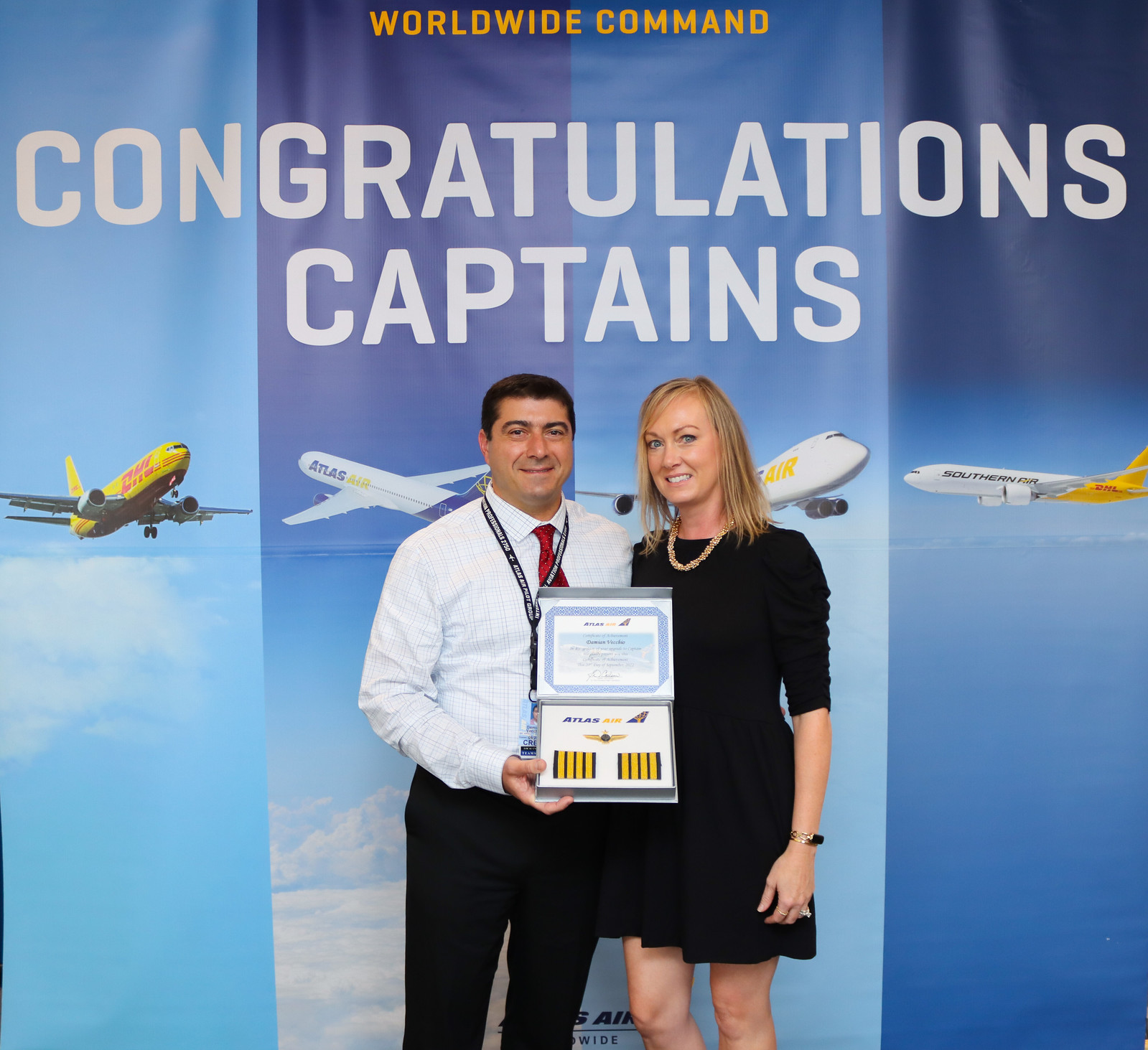In the photograph, a man and a woman, both smiling, are standing side by side in front of a congratulatory backdrop. The man, positioned on the left, is dressed in a white button-down shirt paired with a red tie and black slacks. He has black hair and a name tag necklace around his neck. In his right hand, he proudly holds a certificate adorned with arrow wings. The woman next to him, to the right, wears a black dress and a gold necklace. Her blonde hair frames her cheerful face, and she sports a watch or bracelet on her left wrist along with a ring on her left index finger.

The backdrop behind them is vibrant, featuring bold white letters that read "Congratulations Captains." Four images of airplanes are displayed in a vertical layout with alternating light blue and dark blue categories. From left to right, the airplanes are yellow, white, white, and white with a yellow tail. At the top of the backdrop, the phrase "Worldwide Command" is prominently displayed in yellow lettering.